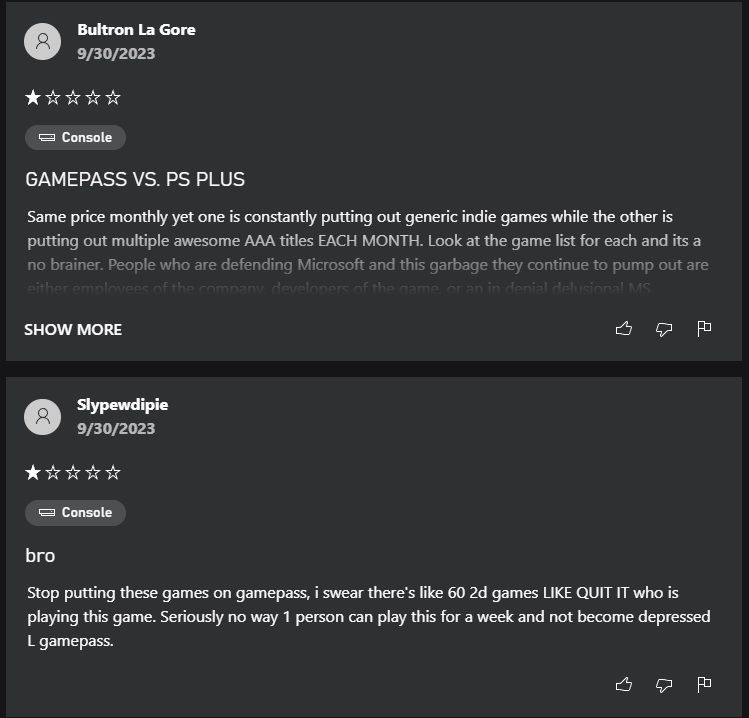A detailed caption for the image of the reviews could be:

---

**Screenshot of Two User Reviews**

The image displays two user reviews for a gaming service, presented as wide rectangular sections stacked vertically.

**Review 1:**

- **User:** Voltron LaGore
- **Date:** 09/30/2023
- **Rating:** ☆★★★★☆ (1 out of 5 stars)
- **Profile Picture:** Blank silhouette with a slight head outline
- **Review Title:** **"Game Pass vs PS Plus"** (all in capital letters)
- **Review Content:** The review starts with a criticism comparing the value of Game Pass to PlayStation Plus, pointing out that though both services are priced similarly, one offers "generic indie games" while the other provides "multiple awesome AAA titles each month." The user emphasizes this comparison by capitalizing "Each month." The review then goes on to criticize those who support Microsoft, suggesting they are either employees, game developers, or "in denial delusional MS." The text fades out here, leaving the remainder of the review unreadable unless the "Show more" option is clicked. 
- **Reaction Icons:** Located on the right side, there are options to give a thumbs up, thumbs down, or report the review with a flag icon.

**Review 2:**

- **User:** Sly Pew Dippy
- **Date:** 09/30/2023
- **Rating:** ☆★★★★☆ (1 out of 5 stars)
- **Profile Picture:** Blank silhouette with a slight head outline
- **Review Title:** **"bro"** (all in lowercase)
- **Review Content:** This brief review expresses frustration with the types of games available on Game Pass, complaining about the abundance of 2D games. The user urges the service to stop adding such titles and questions who enjoys playing them, suggesting that continued play could lead to depression. The review ends with the phrase "Owl Game Pass," which seems to be a typo or autocorrect error for "All Game Pass."
- **Reaction Icons:** Similarly, this review also includes the thumbs up, thumbs down, and flag icons on the far right.